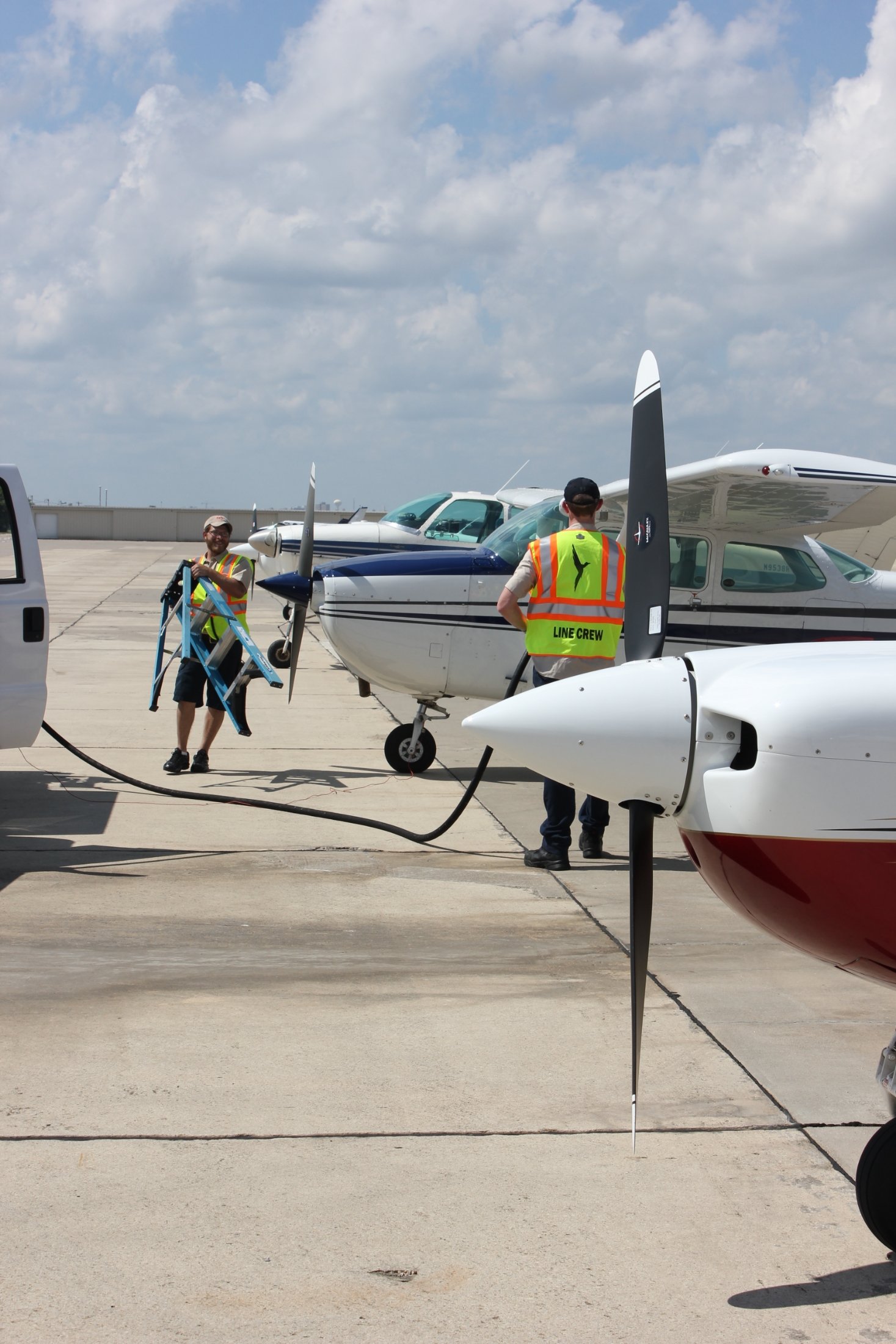In this outdoor airport image, a concrete surface extends into the distance with a large building visible far in the background. The blue sky is mostly obscured by pleasant white-gray clouds. On the right side, three primarily white small passenger airplanes, accented with maroon and blue, stand in a row. Their black propellers are prominently displayed. The left side features a partially visible vehicle, potentially a fueling truck, with an open door and a connected hose leading towards one of the planes. A man in a neon yellow and orange safety vest and a baseball hat is actively fueling the aircraft. Nearby, another man, also wearing a high-visibility vest and a baseball hat, approaches while carrying a blue stepladder. The scene captures a busy moment in the middle of the day, giving a detailed slice of life at an airport.